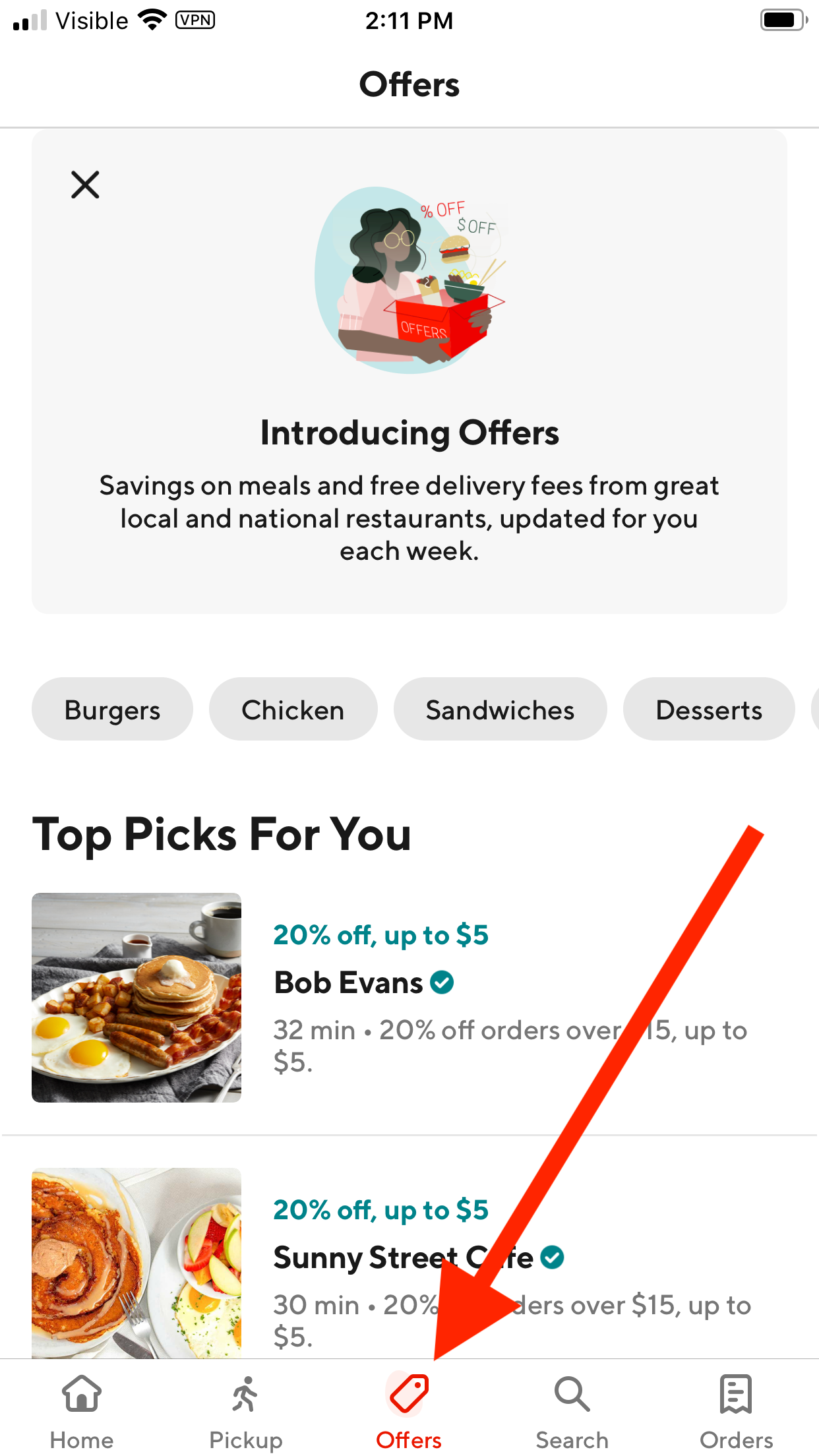This is a screenshot from the "Offers" tab in DoorDash, showcasing a clean and user-friendly interface against a white background. At the top center, the word "Offers" is prominently displayed in black font. Beneath the title, a large grey square dominates the screen with a darker grey square positioned in the top left corner of the larger square. In the center, there is a clipart illustration of a woman carrying a box of takeout. Below this image, "Introducing Offers" is boldly written in black font, followed by a concise description.

Further down, a horizontal scrollable list of categories appears, each encapsulated in grey ovals with black font. The categories include "Burgers," "Chicken," "Sandwiches," and "Desserts." Below this, the heading "Top Picks for You" is showcased in large black font, leading into a vertical list of various offers.

On the right side of the page, a diagonal red arrow points directly at the "Offers" section, highlighting where users can access special deals. At the bottom of the screenshot, a navigation panel is visible, with the "Offers" tab centered and highlighted in red, further emphasizing its importance. The red arrow, pointing at this tab, guides users to click on "Offers" at the bottom to access the special offers page.